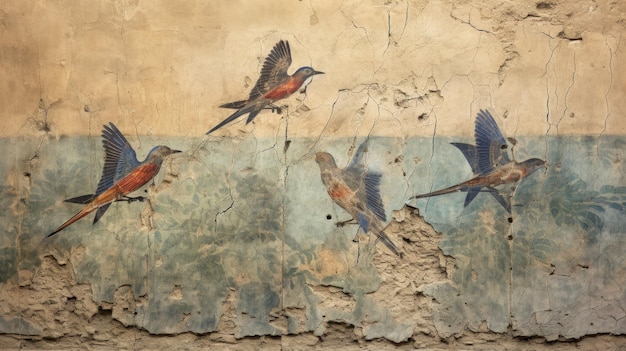This image showcases a highly weathered wall fresco, with evident erosion and chipping at the bottom where the plaster reveals a tan stone or plaster beneath. The fresco's lower half features a muted pastel green evocative of marshland plants. From this marshland, four birds, strikingly detailed with orange breasts and dark wings, emerge in full flight. Two of these birds are positioned toward the bottom left corner, and two are in the top right.

On the right side of the fresco, two other birds of a different kind can be seen. One bird, with dark wings and a tan body, flies off to the right, while another bird, though heavily damaged, is discernible facing the brightly colored birds. The background above the marshland scene transitions to a light blue and dark gray mix, adding a sense of depth, while the fresco's uppermost part remains a plain tan or light brown.

The birds, viewed from a side angle, are richly detailed. They have blue wings with darker flight feathers, an orange breast, a grayish-blue head, and a long tail, making them appear larger than a robin but less heavily marked than a pheasant. The upper area of the fresco, devoid of any imagery, is marked by cracks and pit marks, indicating the fresco's antiquity and the passage of time.